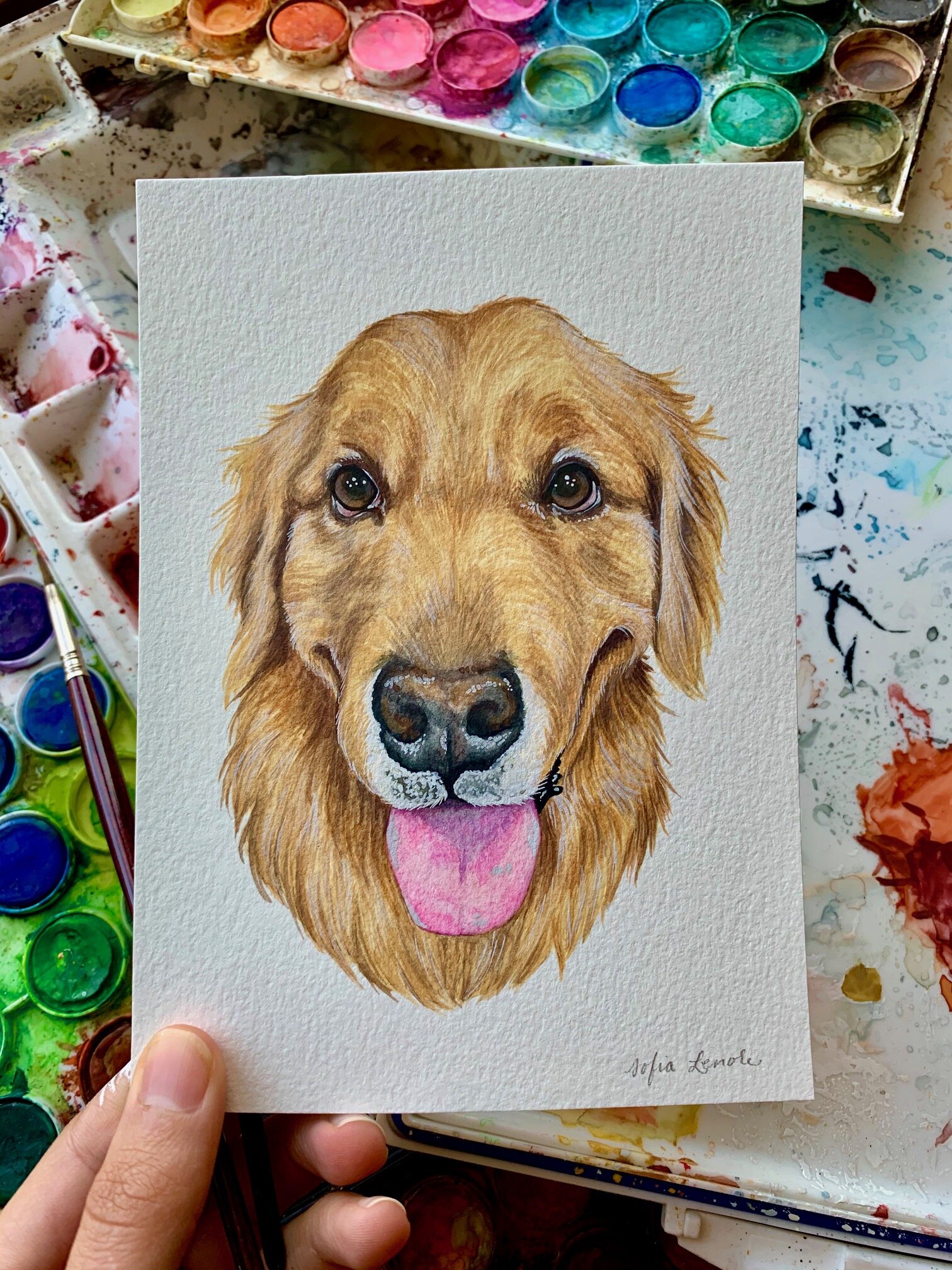In this detailed photograph, we see an artist holding up a small, postcard-sized painting of a golden retriever, hand-drawn with watercolors. The painting captures the head of the dog, characterized by its light brown fur, brown eyes, black nose, and a pink tongue sticking out, giving the dog a cheerful and realistic appearance. The artist, identified as Sophia Lenole by her gray signature in the bottom right-hand corner, holds the artwork delicately between her thumb and index finger of her left hand. Surrounding the painting, the workspace is visible, cluttered with the tools of the trade—various containers of paints in colors like greens, blues, pinks, and reds, as well as an array of paintbrushes and mixing dishes, indicating a vibrant and busy creative process. The background is a rough white texture, which provides a simple contrast to the colorful and detailed painting.